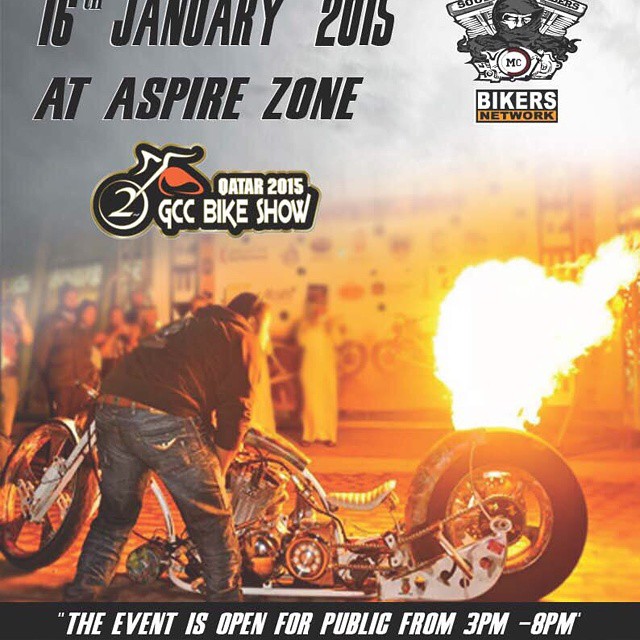This color photograph is an advertisement poster for the 2015 GCC Bike Show, held on 16th January 2015 at Aspire Zone, Qatar. The poster features a vibrant graphic of a red motorcycle with black wheels, alongside branding for the "Bikers Network," which is displayed in black and yellow in the top right corner, incorporating an image of a face between two motorcycle cylinders. Central to the image is a man dressed in a black jacket with a hood and blue jeans, standing over a parked, custom low-rider motorcycle. Behind the man and the bike, a bright orange flame dramatically illuminates the scene. In the background, people, including a woman in a white dress, are visible, captivated by the fiery display. The bottom footer of the poster clearly announces that the event is open to the public from 3 p.m. to 8 p.m., inviting attendees to this outdoor spectacle.